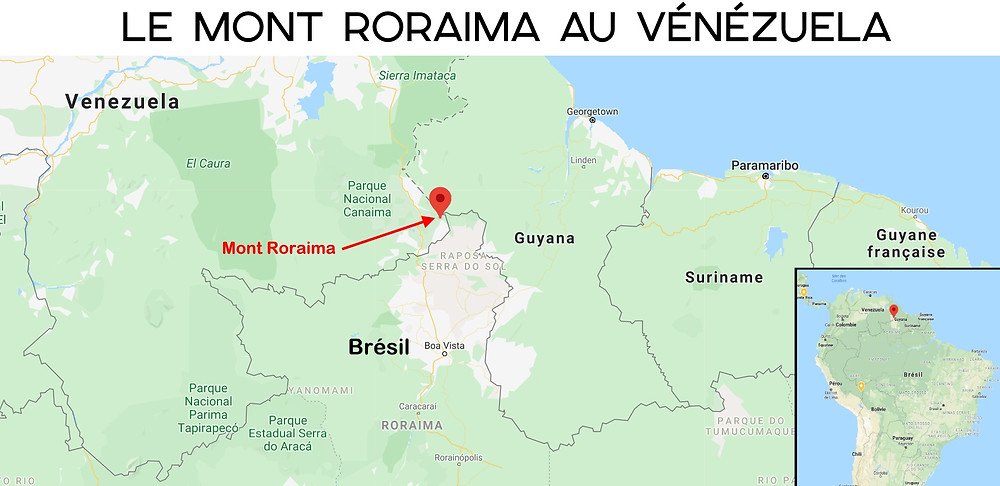This image displays an intricately detailed map with the title "Le Monde, Roraima, Venezuela" prominently placed at the top, indicating the map is in French and is centered around Roraima, a renowned mountain in Venezuela. The map encompasses parts of neighboring countries, including the uppermost section of Brazil and portions of Guyana and Suriname. Highlighted in striking red text is the label "Mount Roraima," accompanied by a red arrow and a pinpoint indicating the exact location of the mountain on the map. Additionally, the map features text identifying "Parque Nacional Canaima," which suggests the inclusion of the Canaima National Park, a significant national park in Venezuela known for its natural beauty and geographical landmarks. The detailed cartography, along with textual annotations, collectively provides a comprehensive geographical context of the region surrounding Mount Roraima.